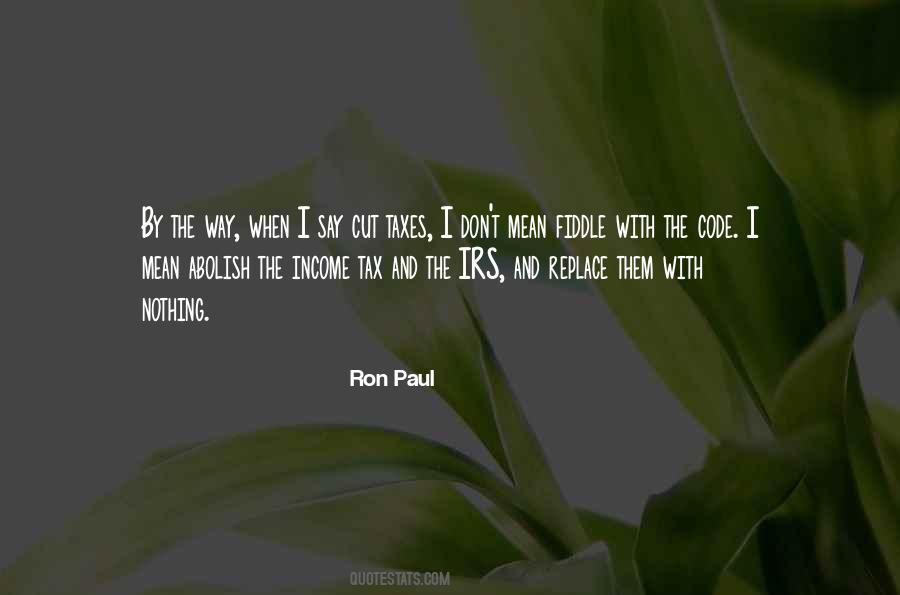The image features a darkened background with green leaves, resembling a house plant, against a gray tone. Sunlight filters through, but the overall effect is subdued by a grayscale overlay. Centered on the image is a quote in white text, saying, "By the way, when I say cut taxes, I don't mean fiddle with the code. I mean abolish the income tax and the IRS and replace them with nothing." Beneath this quote, in white font and all uppercase letters, it reads, "Ron Paul - QUOTESTATS.COM." The strong, centered text contrasts with the dark, plant-filled background, making the quote stand out prominently.